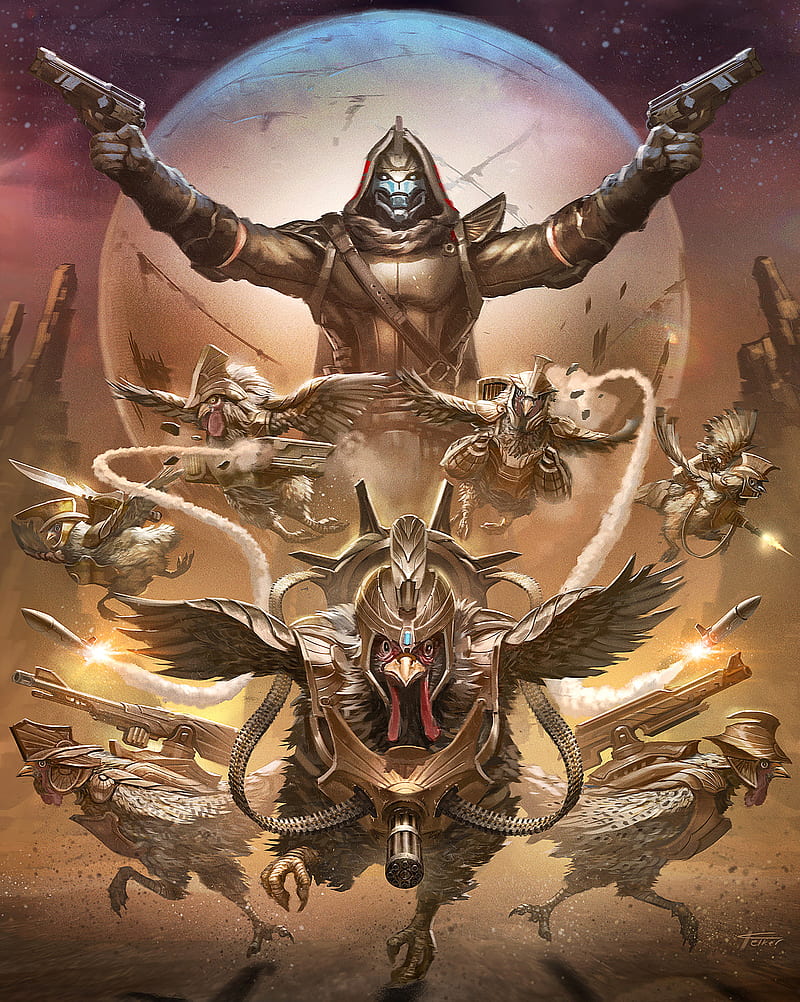This captivating science fiction scene showcases an intriguing blend of organic and mechanical elements, centered around a group of armored, weapon-wielding chickens. At the heart of the tableau is a menacing, cloaked robotic figure, arms spread wide as it brandishes a gun in each hand. The figure stands against the backdrop of a vast, round planetary shape, likely indicating an alien world or an interstellar setting.

In the foreground, two chickens wearing elaborate armor and helmets soar through the air, each heading in opposite directions, exuding a sense of dynamic movement and urgency. Below this aerial duo, two more chickens can be seen, each positioned on either side of the frame, armed and ready for battle with weapons mounted on their backs.

Dominating the lower central part of the image is a larger, imposing chicken, advancing directly towards the viewer with a sense of determined purpose. Flanking this central figure, two additional chickens are depicted in profile, each equipped with headgear and back-mounted weapons, adding to the overall militaristic and futuristic atmosphere.

The detailed armor and weaponry of the chickens, combined with the presence of the sinister robotic figure and the planetary backdrop, create a rich, imaginative scene that invites viewers to ponder the narrative and world-building behind this unique science fiction tableau.